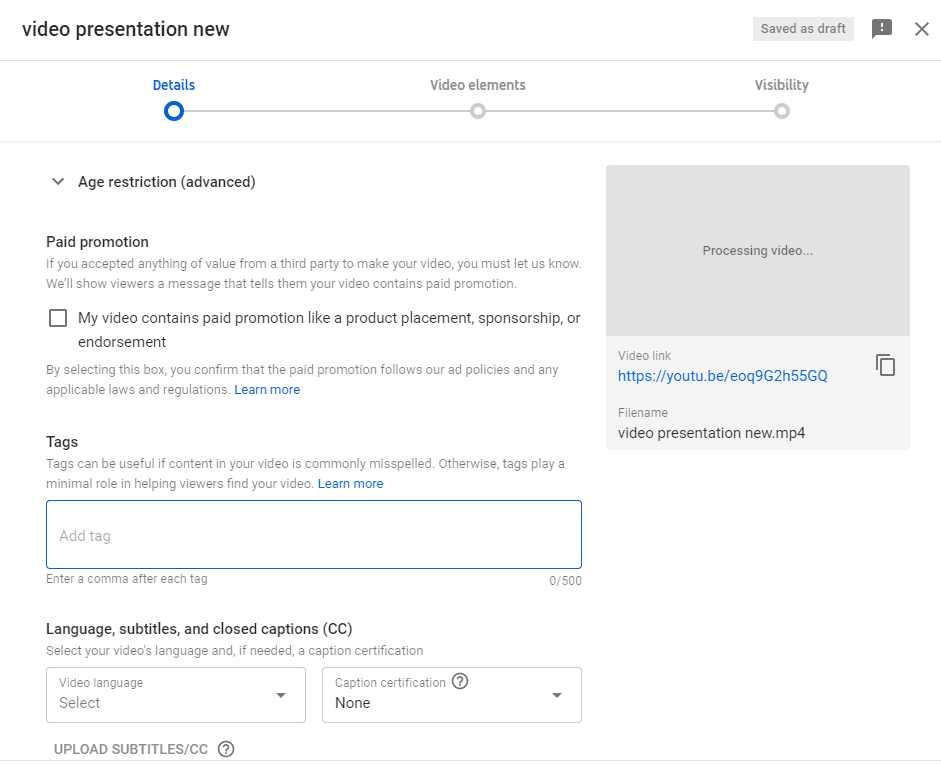**Detailed Description of the Screenshot:**

The image is a screenshot of a web page with a predominantly white background, featuring mostly gray and blue text. The layout is simple and plain. At the top of the page, there is a banner. On the left side of the banner, the text "Video Presentation New" is displayed. On the right side of the banner, there are three elements: a “Saved as Draft” button, an exclamation point icon, and an "X" button.

Directly below this banner is a horizontal slider bar with three labeled sections: "Details," "Video Elements," and "Visibility." The "Details" section, situated on the far left, is highlighted with a blue circle and blue text, indicating it is the active section.

Beneath the slider, the content is divided into two main columns. On the right side, underneath the "Visibility" label (found directly beneath the banner), there is a gray rectangle with the text "Processing Video" centered inside. Below this rectangle, a video link and file name are displayed.

On the left side of the page, the content starts with an "Age Restriction" heading, followed by an advanced scroll arrow. Below it is a "Paid Promotion" section. This section includes a brief explanatory text and an unchecked box labeled "My video contains paid promotion like a product placement, sponsorship, or endorsement."

Following this is a "Tag" section. There is an input box outlined in blue that prompts to "Add Tag." 

In the bottom left corner of the screenshot, there is a heading titled "Language, Subtitles, and Closed Captions." This section contains dropdown boxes for selecting "Video Language" and "Caption Certification." Beneath these, the text "Upload Subtitles / CC" is accompanied by a question mark enclosed in a circle, indicative of additional help. A thin gray line separates this section from the rest of the content.